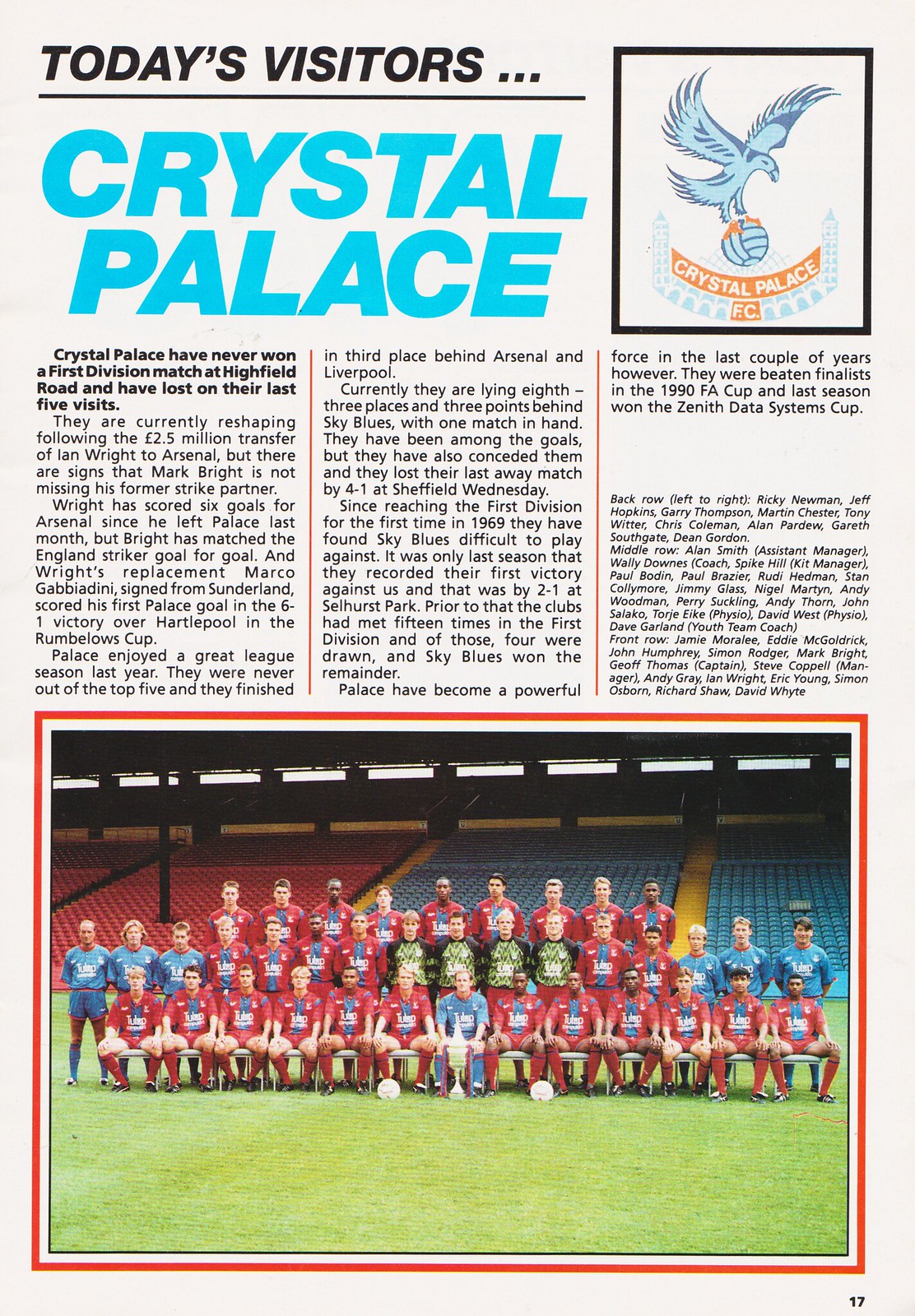The image is a detailed page from a soccer magazine, centered around the visiting team, Crystal Palace. Positioned prominently at the top, the headline reads "Today's Visitors: Crystal Palace," accompanied by the team's logo in the top right corner. The logo features a bird with outstretched wings perched on a soccer ball, with "Crystal Palace" inscribed below it. The primary text begins with, "Crystal Palace have never won a First Division match at Highfield Road and have lost on their last five visits," followed by several paragraphs of detailed information about the team's history and performance.

Covering the bottom half of the page is a large, comprehensive photograph of the Crystal Palace team. The team is arranged in three distinct rows: the front row of players is seated, the middle row is standing, and the back row stands elevated on stools. Most of the players don red jerseys, while a few are in blue, indicative of a mix in their uniforms. Additionally, there are four to five individuals in black or green jerseys, likely the coaches. The team poses with a trophy prominently displayed in the center, and soccer balls scattered on the field, suggesting a celebratory moment. In the backdrop, rows of stadium seating can be discerned, completing the setting.